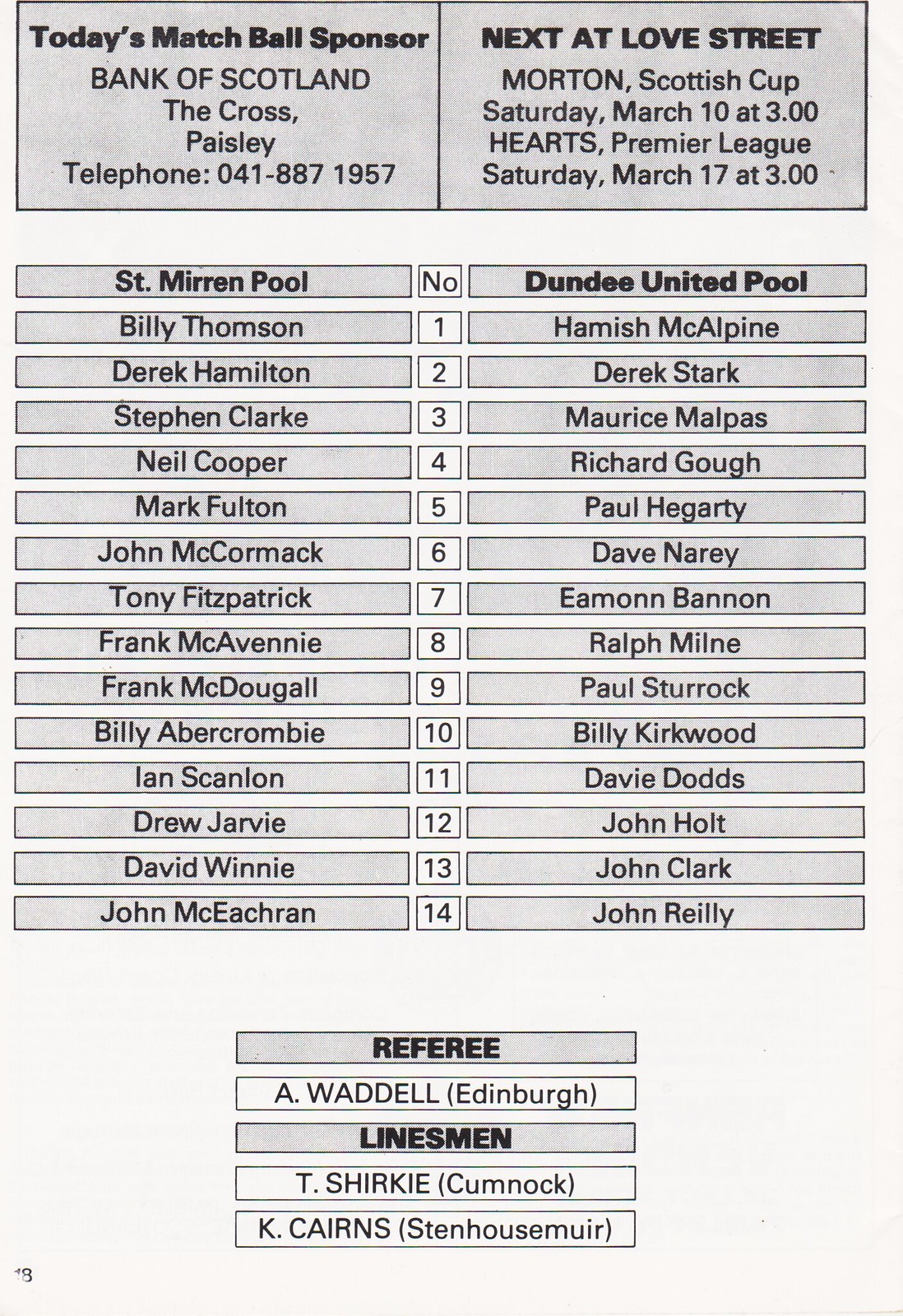This image is a tall rectangular page from a sports catalog or game day program, set against a light grey background. At the top, a darker grey rectangular banner, divided into two sections by a black line, features advertisements. The left section reads in black text, "Today's Matchball Sponsor: Bank of Scotland, Lacrosse, Paisley, Telephone 041-887-1957." The right section announces upcoming events with the text, "Next at Love Street: Morton, Scottish Cup, Saturday, March 10th at 3; Hearts, Premier League, Saturday, March 17th at 3."

Below these advertisements, a central column numbered 1 through 14 divides the page into two lists. The left list is titled "St. Mirren Pool" and includes names such as Billy Thompson, Derek Hamilton, Stephen Clark, Neil Cooper, and Mark Fulton, continuing down to John McCarron at number 14. On the right, the list titled "Dundee United Pool" features names like Hamish McAlpine, Derek Stark, Maurice Malpas, and Richard Gough, ending with John Riley at number 14.

At the bottom of the page, the officials for the match are noted: the referee is A. Waddell from Edinburgh, and the linesmen are T. Shirky from Cumnock and K. Cairns from Stenhousemuir. The page is printed in black and white, with the page number indicated as 18 at the bottom left corner.